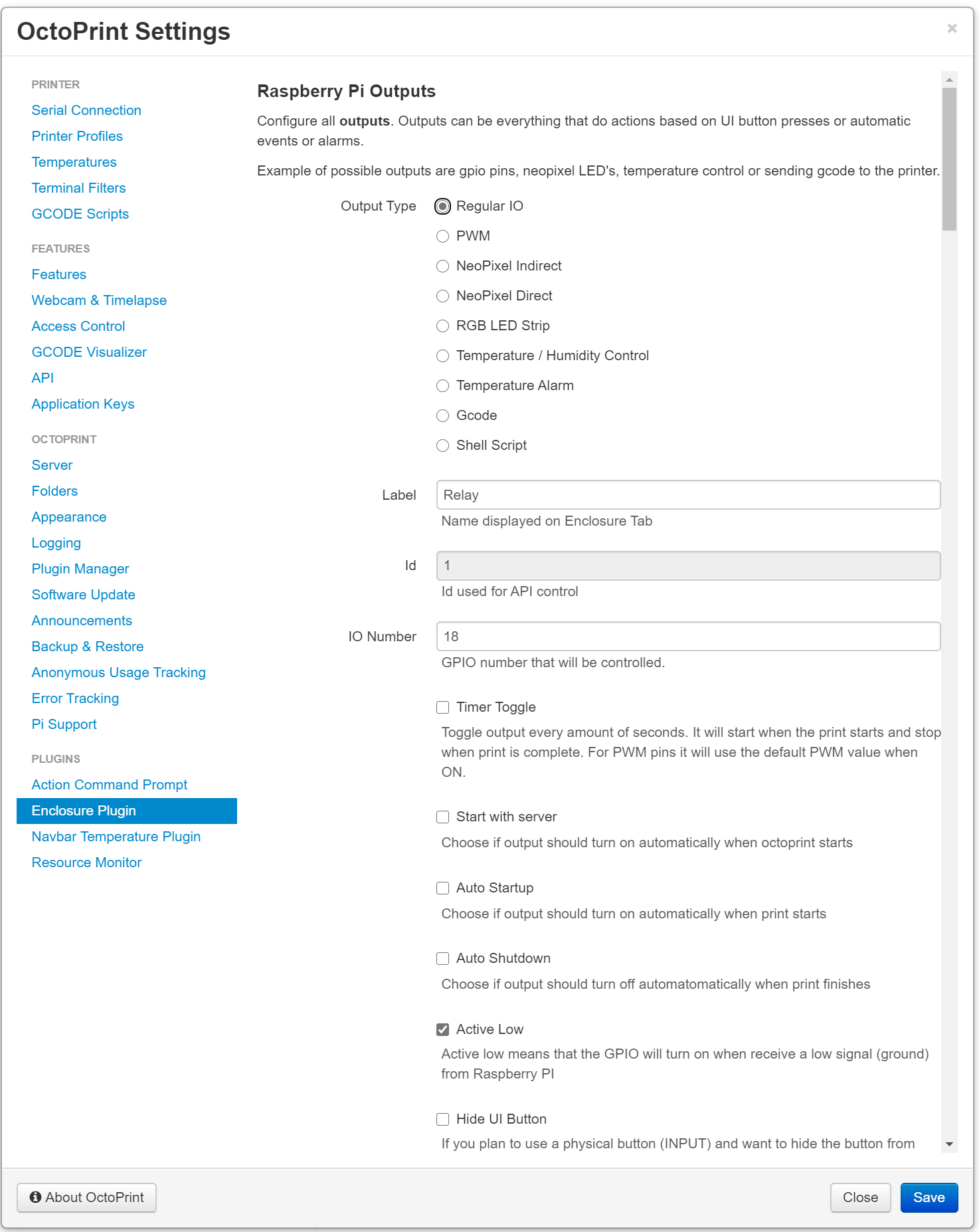The image displays the settings page for OctoPrint, showcasing an organized interface with multiple configuration options.

**Upper Section:**
- **Top Left Corner:** The header "OctoPrint Settings" is displayed, followed by a horizontal gray line.
- **Top Right Corner:** There is a light gray 'X' button, presumably to close the settings window.

**Left Sidebar:**
- **Categories and Options:** The sidebar lists different categories, each with several sub-options:
    - **PRINTER** (Gray, capitalized):
        - Serial Connection
        - Printer Profiles
        - Temperatures
        - Terminal Filters
        - G-Code Scripts
    - **FEATURE** (Gray, capitalized):
        - Features
        - Webcam & Time-Lapse
        - Access Control
        - G-Code Visualizer
        - API
        - Application Keys
    - **OCTOPRINT** (Gray, capitalized):
        - Server
        - Folders
        - Appearance
        - Logging
        - Plugin Manager
        - Software Update
        - Announcements
        - Backup & Restore
        - Anonymous Usage Tracking
        - Error Tracking
        - Pi Support
    - **PLUGINS** (Gray, capitalized):
        - Action Command Prompt
        - Enclosure Plugin (currently focused, highlighted with a dark blue box)
        - Navbar Temperature Plugin
        - Resource Monitor

**Main Section (Focused on Enclosure Plugin):**
- The section is dedicated to setting up the Enclosure Plugin, with a header "Raspberry Pi Outputs" in bold.
- Below the header, there's a description outlining the configuration of various outputs. Outputs include GPIO pins, NeoPixel LEDs, temperature controls, and sending G-Code to the printer.

**Configuration Options:**
- **Output Type:** A series of radio buttons including:
    - Regular IO (selected)
    - PWM
    - NeoPixel Indirect
    - NeoPixel Direct
    - RGB LED Strip
    - Temperature/Humidity Control
    - Temperature Alarm
    - G-Code
    - Shell Script
- **Label:** A text box filled with "relay," indicating the name displayed on the enclosure tab.
- **ID:** A grayed-out box with the number "1," used for API control.
- **IO Number:** A box with "18" indicating the GPIO number to be controlled.

**Checkbox Options:**
- **Timer Controlled Toggle:** Not checked, with an explanation that it toggles output every set amount of seconds during a print job.
- **Start with Server:** Not checked, decides if the output should turn on when OctoPrint starts.
- **Auto Setup Startup:** Not checked, decides if the output should turn on when a print starts.
- **Auto Shutdown:** Not checked, decides if the output should turn off when a print finishes.
- **Active Low:** Checked, meaning the GPIO will turn on with a low signal.
- **Hide UI Button:** Not checked, the text is partially cut off, but it implies hiding the button for physical input usage.

**Bottom Section:**
- The left side features an "About OctoPrint" button with an information icon.
- The right side includes two buttons:
    - **Save:** Blue with white text (currently focused).
    - **Close:** Gray with black text.

This detailed caption highlights all the elements and their functions, offering a comprehensive understanding of the image's content.